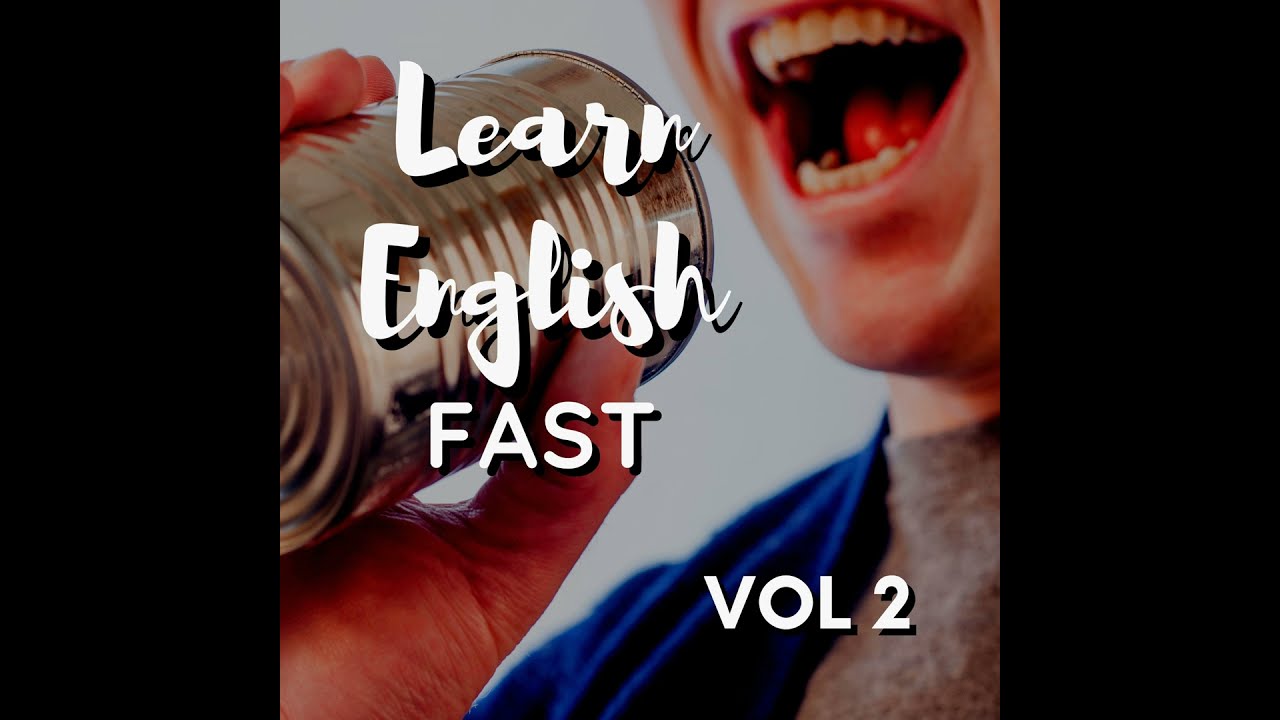The image depicts the cover of a learning book titled "Learn English Fast, Volume 2." It features a close-up of a white male speaking into a shiny, silver tin can. The man's mouth is wide open, showcasing both his top and bottom teeth, and his tongue is visible. His face is partially shown, focusing mainly on his mouth, with just the sides of his face included. He is dressed in a gray shirt beneath a blue jacket or pullover. His hand holds the tin can up to his mouth as if he is singing or talking into it, reminiscent of the childhood game where a string-connected can transmits sound to a distant listener. The text "Learn English Fast" is written in a unique, cursive white font with black drop shadows, while "Volume 2" appears in a standard blocky font, also white with black drop shadows. The background is predominantly white with two black vertical columns on the right side, lending a humorous and educational vibe to the image.